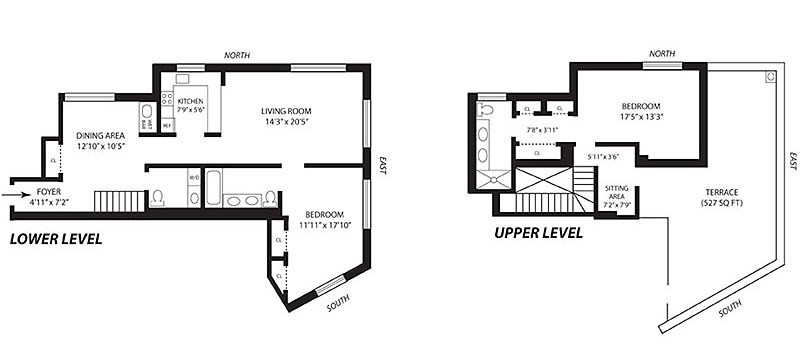This image showcases a detailed set of blueprints for a two-bedroom house. Upon entering the lower level through the foyer, you are greeted by a stairway directly in front of you leading to the upper floor. Turning left from the foyer, you enter the dining area. Continuing through, you arrive at a compact kitchen, measuring just 7.9 by 5.6 feet. A powder room is conveniently located beneath the stairs. Adjacent to the kitchen lies a spacious living room, measuring 14.3 by 20.5 feet.

Connected to the living room is a bedroom measuring 11.11 by 17.10 feet, which features two closets and a private en suite bathroom, adding both functionality and privacy.

Ascending to the upper level, another bedroom awaits, measuring 17 by 13 feet. This floor also features a cozy sitting area. The upper-level bathroom is designed with a shower and a double vanity, indicating that it is likely the master bathroom. Additionally, this level offers access to a terrace, providing an outdoor space for relaxation. The thoughtful layout of the blueprints ensures efficient use of space while maintaining a comfortable living environment.